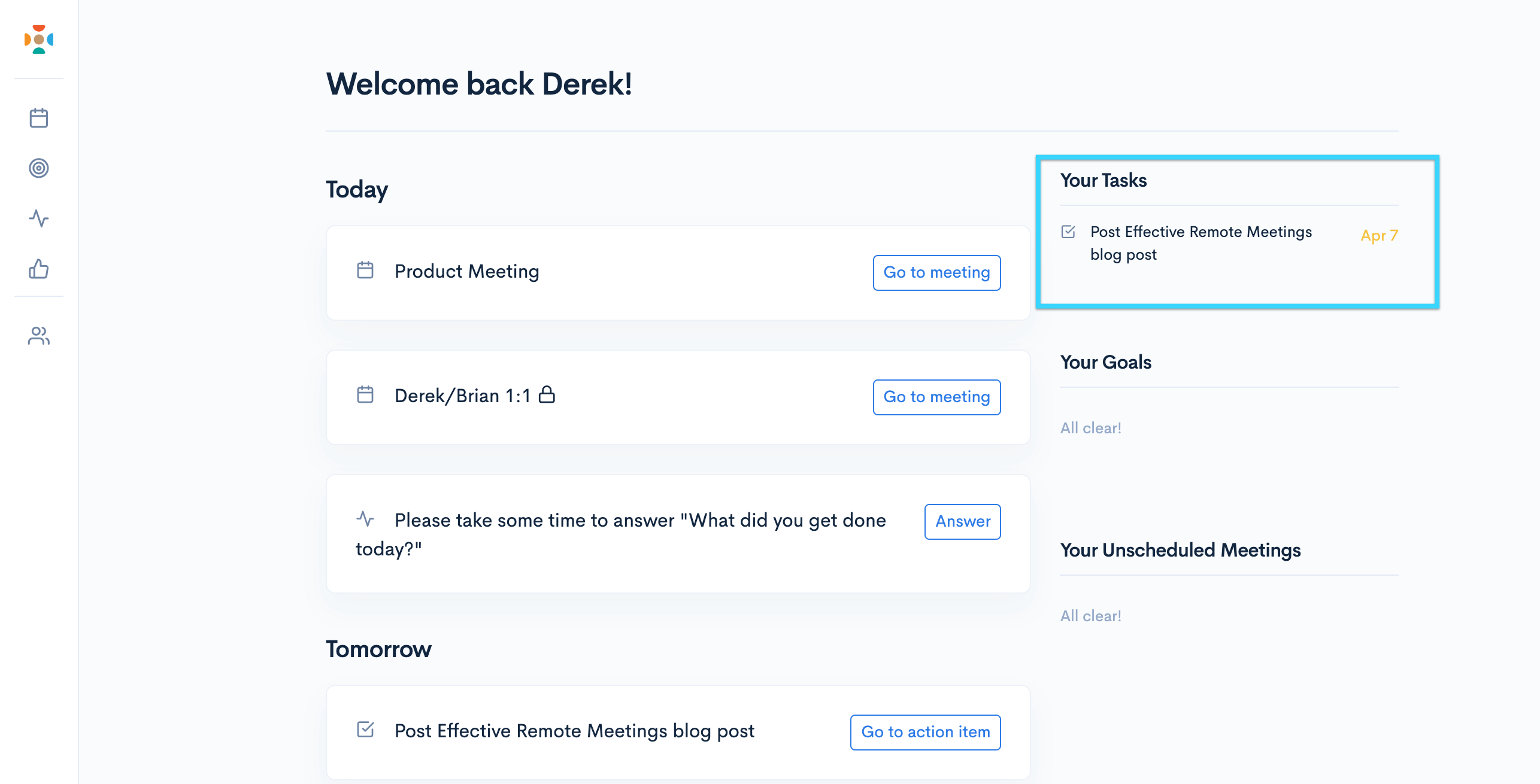In the provided image, a website screen is displayed, prominently featuring personalized user interface elements. At the top left corner, there's a welcoming message, "Welcome back, Derek!" Below this greeting, the heading "Today" is presented, followed by three main sections displayed within white rectangles. 

1. The first section is labeled "Product Meeting," accompanied by a button on the right side that says "Go to Meeting."
2. The second section details a "Derek/Brian One-on-One" meeting, also with the "Go to Meeting" button on its right.
3. The third section prompts the user with, "Please take some time to answer: What did you get done today?" featuring an "Answer" button to the right.

At the bottom of the "Today" section, there is another heading titled "Tomorrow," with a single noted task: "Post effective remote meetings blog post." Next to this task, there's a blue button labeled "Go to Action Item." 

Further down, under a distinct blue rectangular heading labeled "Your Tasks," it highlights the task "Post effective remote meetings blog post," along with an orange date marker indicating "April 7th." Below this section is another heading titled "Your Goals" displaying "All clear" and a final section labeled "Your Unscheduled Meetings," which also reads "All clear."

The entire background of the interface is in light gray. Additionally, at the very top left corner of the screen, there is a colorful icon resembling a plus sign made up of blue, red, green, and yellow segments, reminiscent of common tech icons. Directly beneath this icon are five smaller, gray icons arranged vertically, one below the other.